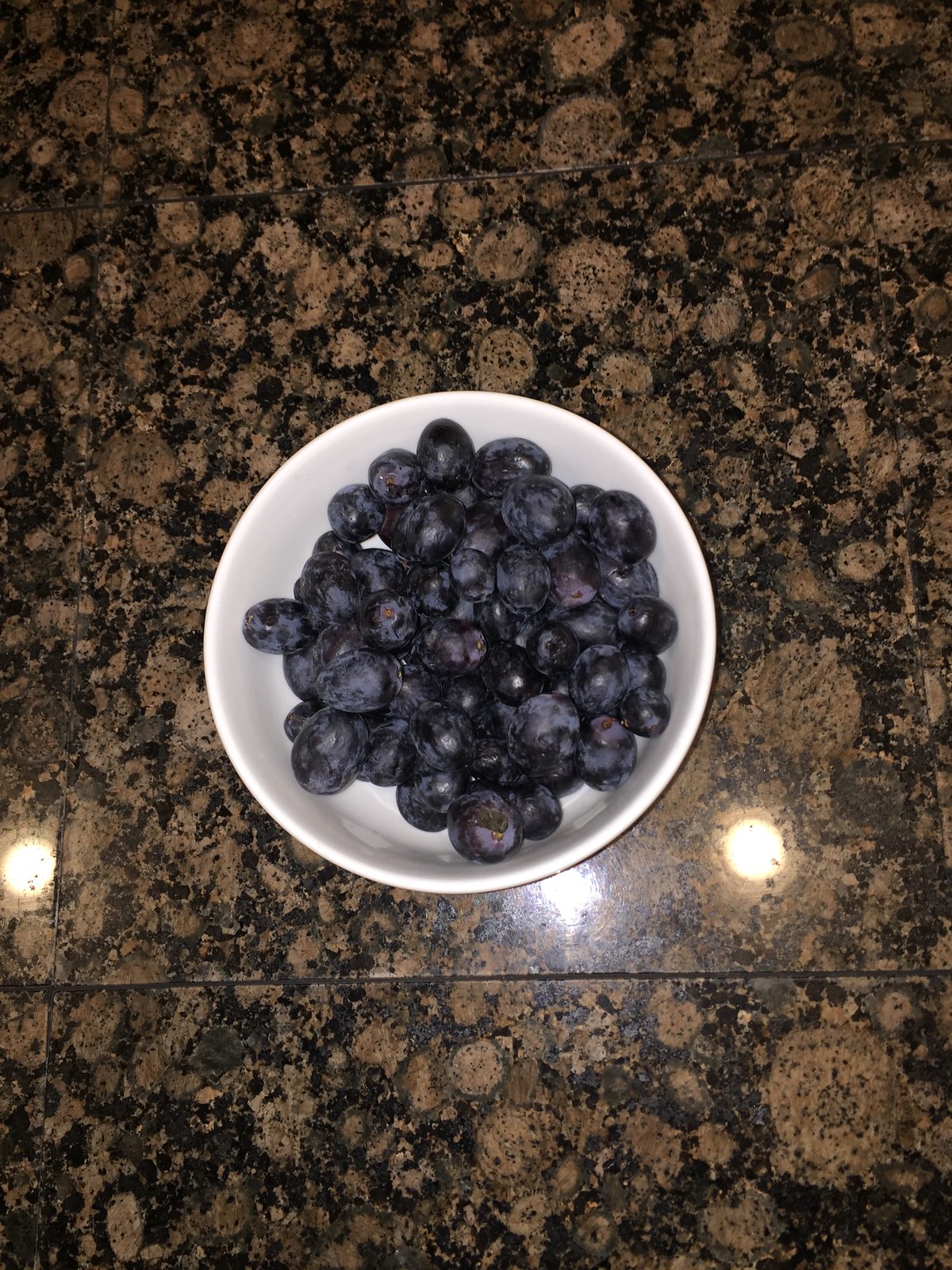This is a vertical, rectangular photograph showcasing a centrally-located white dish brimming with dark, plump blueberries, which are dusted with a light waxy powder. The dish is placed on a shiny granite countertop that features a natural tile look with black, brown, and gold speckles. You can also see little dots of light reflecting off the countertop, suggesting downed ceiling lights on either side. The overall texture and colors of the surface add a rich visual dimension to the composition, with the lights enhancing the reflective quality of the granite.